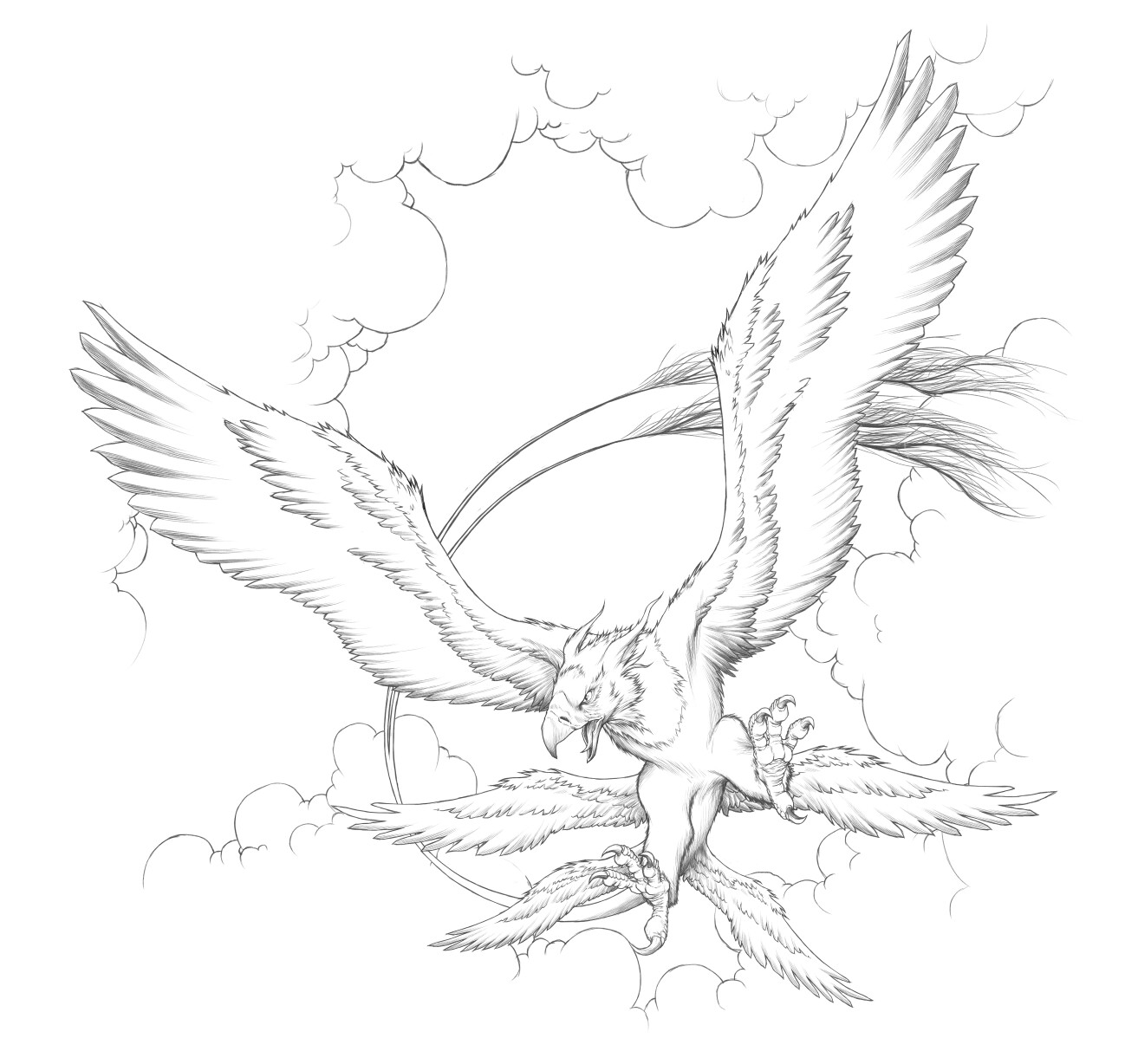The image is a highly detailed black-and-white drawing of an enormous, aggressive bird soaring in the sky. The bird, resembling a griffin, has its menacing eyes fixated downward and its beak wide open, revealing a ferocious expression. Its enormous wings, significantly larger than its body, are outstretched, showing powerful feathered limbs ready to strike. Both sets of talons are open wide as if poised to snatch prey, with sharp, elongated claws on full display. The background features a bright, well-lit sky filled with clouds, drawn with crisp black outlines on a white expanse. Adding to the fantastical nature of the creature, its long, mammalian tail curls in a C-shape behind it, ending in a furry tip. Intriguingly, the bird appears to have extra sets of smaller wings sprouting from its tail area, suggesting a mythical or otherworldly origin. The overall clarity of the image is sharp and detailed, capturing the scene vividly and enhancing the dramatic, tense atmosphere.